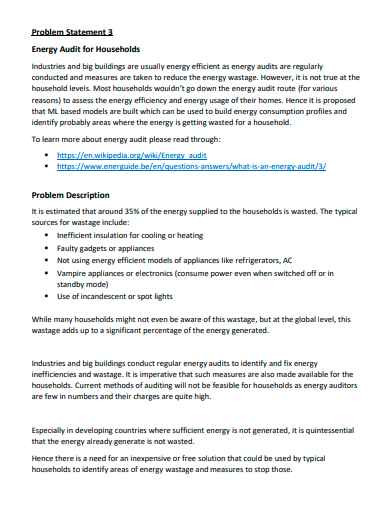### Detailed Caption:
The image displays a meticulously organized problem statement written in black text on a clean white background. This document is formatted like an outline and begins with the underlined heading "Problem Statement 3: Energy Audit for Households." It elaborates that while large buildings and industries often conduct energy audits to enhance efficiency, such practices are rare at the household level. The text argues that households are generally reluctant to pursue energy audits for various reasons, preventing them from assessing their energy efficiency.

The document proposes the development of machine learning (ML)-based models to create household energy consumption profiles, thereby identifying potential areas of energy wastage. To illustrate this point, the text references two external links: "Wikipedia Energy Audit" and "Energy Guide B: Questions and Answers with the Energy Guide Audit."

The next section, titled in bold as "Problem Description," estimates that around 35% of household energy supply is wasted, listing common causes for this inefficiency. The points include insufficient insulation, use of non-energy-efficient gadgets, and the presence of "vampire appliances" that continually draw power. 

The concluding paragraphs emphasize the significant cumulative impact of household energy wastage on a global scale. They highlight the contrast with industries and large buildings that regularly conduct energy audits and implement efficiency measures. Particularly in developing countries, where energy supply is often inadequate, reducing wastage is crucial. The document concludes by stressing the need for an affordable or free solution that households could use to identify and mitigate energy inefficiency.

Overall, the problem statement calls for innovative and accessible methods to help households become more energy-efficient, ultimately contributing to a global reduction in energy wastage.